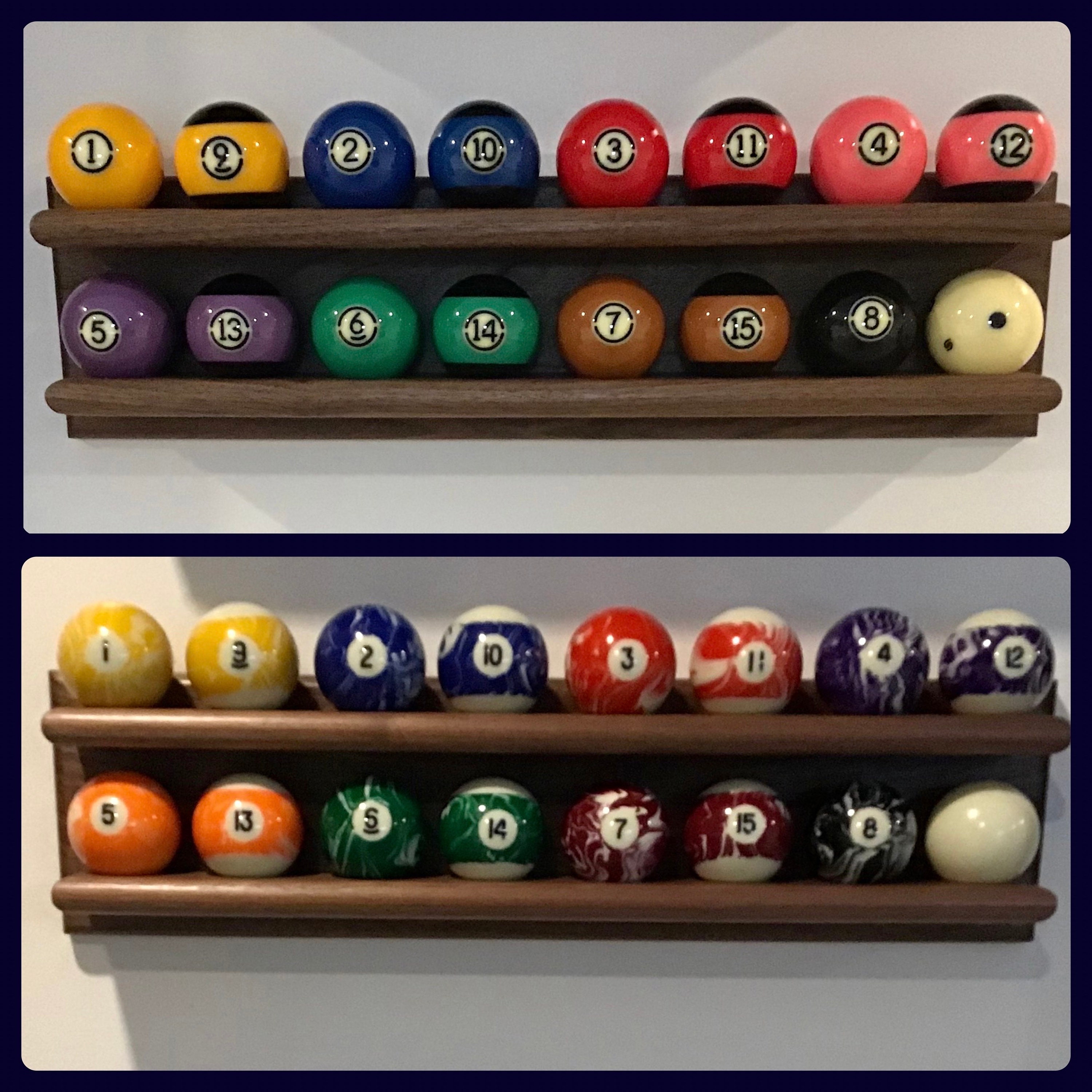The image displays two shelves, each holding a set of pool balls, against a white wall and framed by a black border. Each set is organized by color and features both solid and striped balls. The top row showcases vivid, bold colors, including two of each: yellow, blue, red, pink, purple, green, brown, a black 8-ball, and a cue ball with one black dot. Notably, the colors are very saturated and clear.

In contrast, the bottom row of pool balls has a more distressed, marbled appearance, featuring similar colors but with added white speckles and marbled lines. This set includes yellow, blue, red, purple, orange, green, maroon, a black 8-ball, and a solid white cue ball. Both rows are arranged on brown wooden shelves, with the bottom shelf being darker and more polished compared to the rough, slightly unfinished appearance of the top shelf. Each ball in the top set has a black circle with a white interior, while the bottom set lacks these black outlines, contributing to its distressed look.